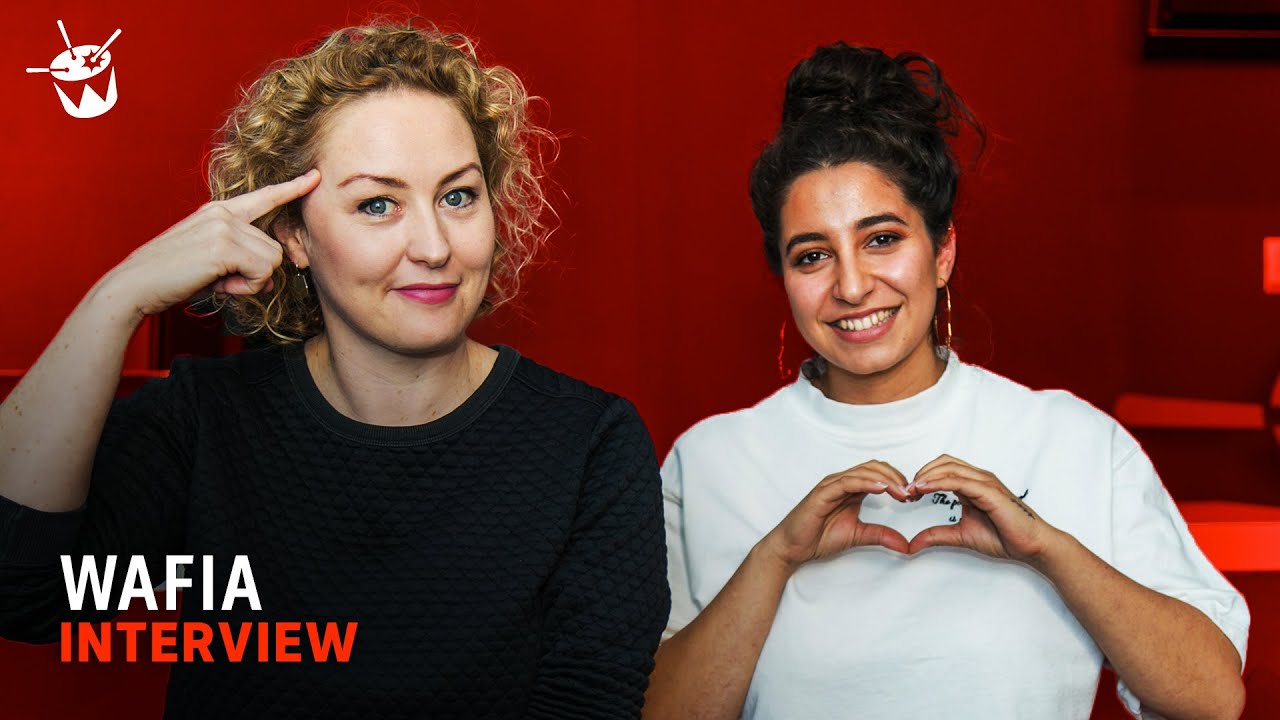This screenshot captures an image displayed on a digital screen, either a computer or phone. The picture features two women posing against a primarily red backdrop. The woman on the left, who is Caucasian with striking blue eyes and brownish, dyed blonde hair, is dressed in a black shirt. She is posing with her head resting on one hand, pointing her finger towards her temple. The woman on the right appears to be of Indian descent, with long black hair and brown eyes. She is wearing a white shirt and is forming a heart symbol with her hands.

Both women are accessorized with earrings; the Indian woman is adorned with large hoop earrings, while the Caucasian woman sports smaller earrings. The upper left corner of the image features a white graphic of a drum being played by three drumsticks. Text overlays the image: "WAFIA" in white letters and "INTERVIEW" in red letters. The overall composition suggests an interview or media feature, accentuated by the vibrant red background that adds an energetic tone to the image.